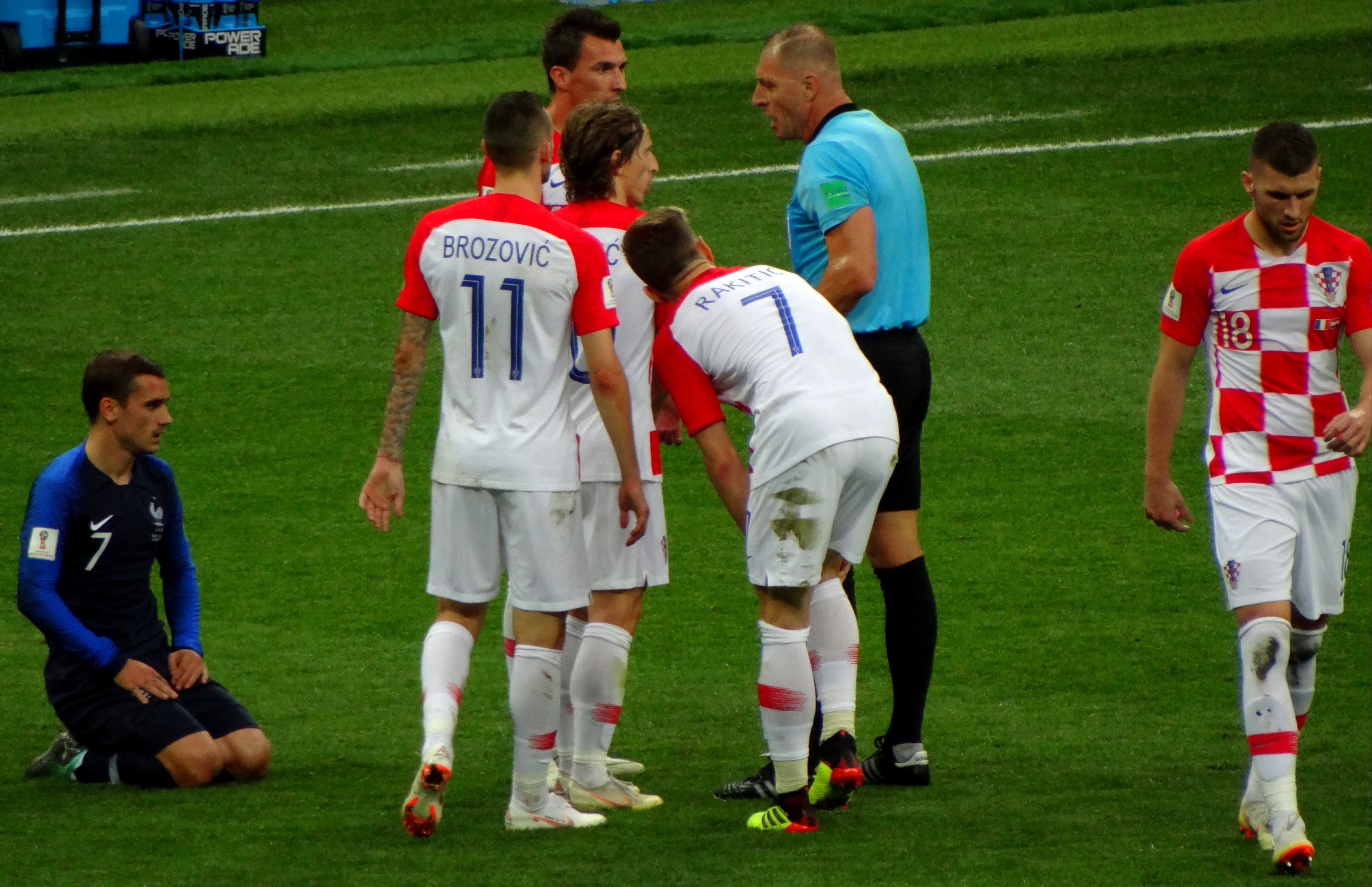In this outdoor image, set on a flat, grassy soccer field, a scene from an intense soccer match unfolds. The center of the image is dominated by a group of seven men, seemingly engaged in a heated argument with a referee dressed in a blue shirt, black pants, and black socks. Four of these players, identified by their red and white jerseys, white shorts, and white socks, belong to the same team. Among them, one player wears the jersey number 11 with the name "Brozovic," while another sports jersey number 7. Off to the left, a player in a blue and black uniform, also wearing number 7, is seen kneeling. To the right, a man in a checkered red and white shirt with white shorts is walking away from the commotion. In the background, a Powerade advertisement is visible, adding a splash of commercial presence to the vivid scene. The field is marked with distinct white lines typical of a soccer field, with the predominant colors in the image being green, white, blue, gray, red, light blue, and light green.